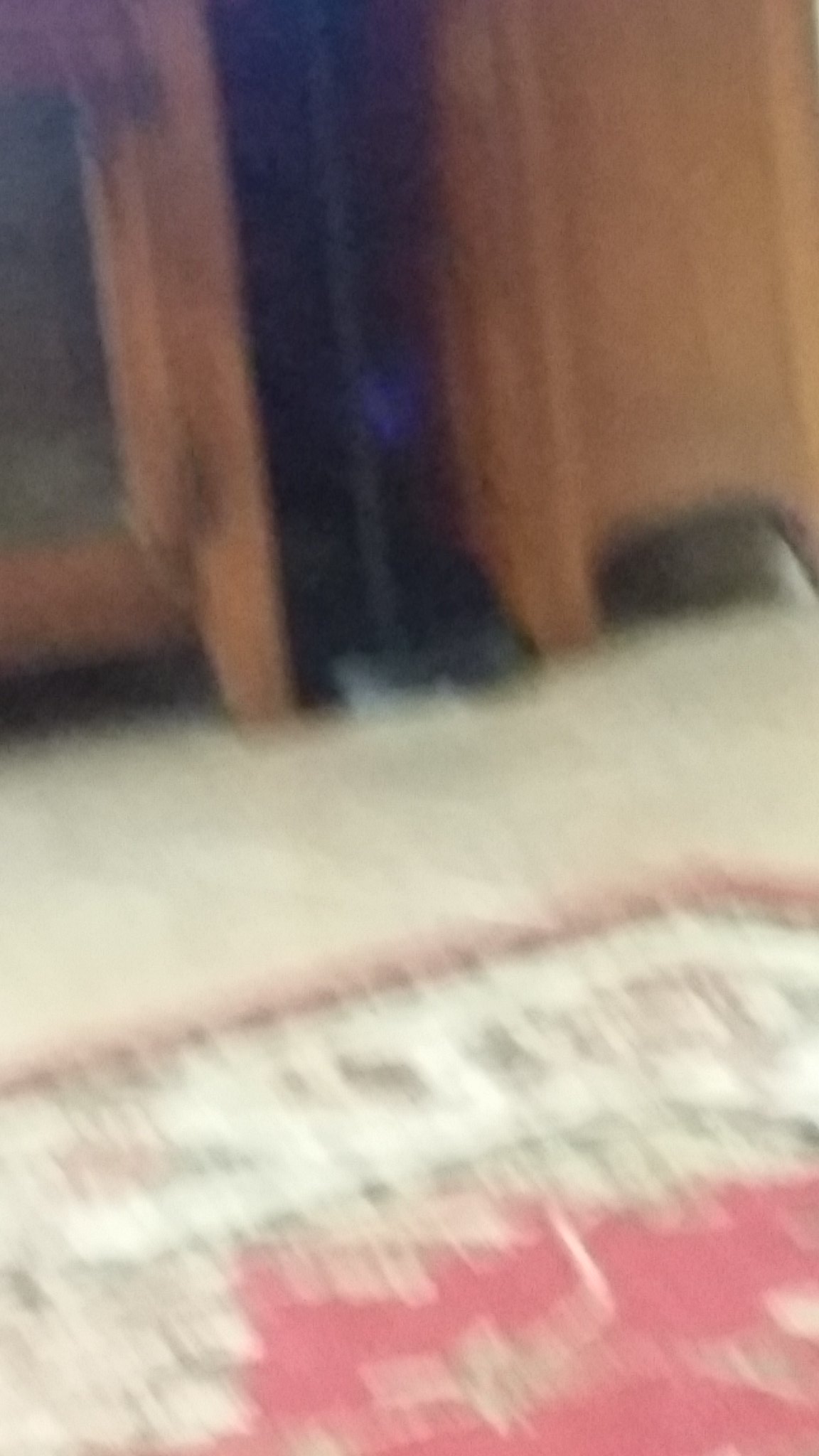This image depicts a blurry indoor scene, likely inside a house. The foreground showcases a light-colored, possibly beige tile or linoleum floor. At the bottom of the image is an ornate red carpet with a white floral pattern and several additional borders, including a thinner brown and red one. In the background, there are two wooden pieces of furniture, possibly dressers, with visible brown legs and glass doors. Between these furniture pieces is a dark gap containing an indistinct black object, which might be a floor lamp or a vacuum cleaner, distinguished by a faint blue element and a gray line resembling a pole or handle. Overall, the image suffers from poor focus, making specific details challenging to discern.